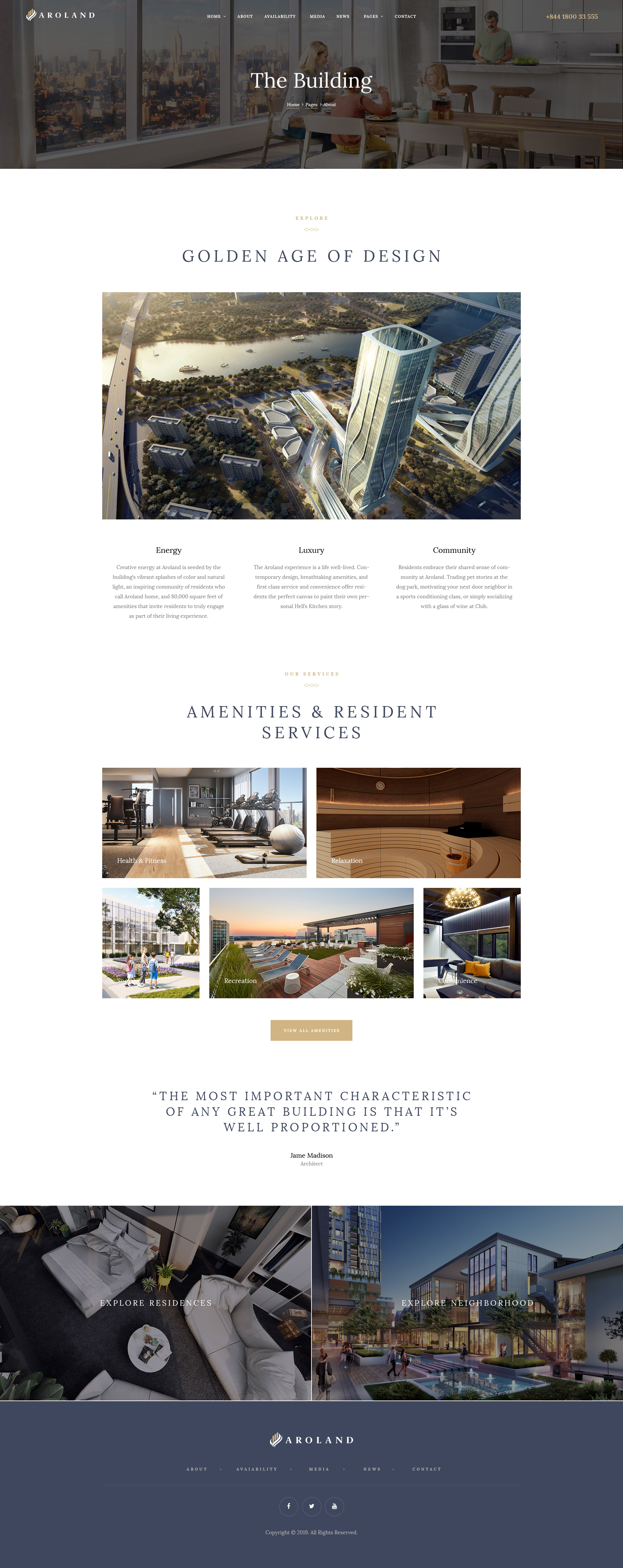This image appears to be a screenshot from a tablet showcasing a website design or advertisement for a company that manages or rents out apartments and condos in a high-rise building in a major city. The website features a sophisticated layout with a predominantly gray header, which carries a slightly transparent overlay. Prominent white text within the header reads, "The Building: Golden Age of Design."

The website seems to focus heavily on visual content, displaying a series of colorful, well-curated images in a long, scrolling format. These images likely highlight various apartments, amenities, and resident services offered by the company. Various sections can be identified, including menus for amenities, resident services, and more.

Further down the page, additional sections seem to provide detailed information about the company, such as an "About Us" section, contact information, and options for virtual tours. The color palette of the website is subtle and polished, featuring harmonious shades of browns, blues, and golden yellows, contributing to an overall sense of elegance and modernity.